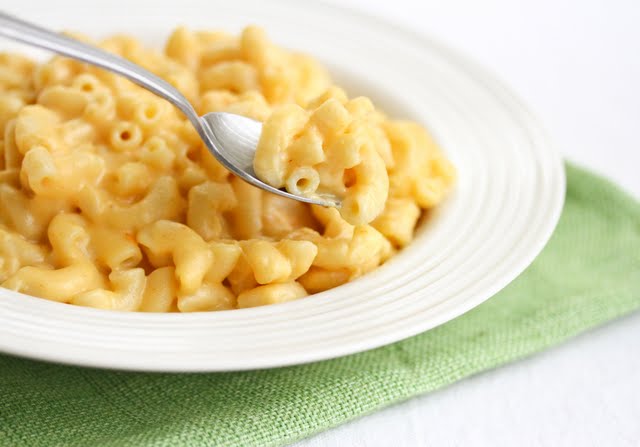The image is a rectangular photograph depicting a plate of macaroni and cheese. The pasta is elbow-shaped and covered in a rich, orange-colored cheese sauce. The macaroni is presented on a shallow, white porcelain plate with a wide rim. A metal spoon filled with a portion of the macaroni and cheese hovers above the plate, positioned near the top-left corner. The plate is set on a green canvas placemat which rests on a white table. The overall presentation looks appetizing and inviting.